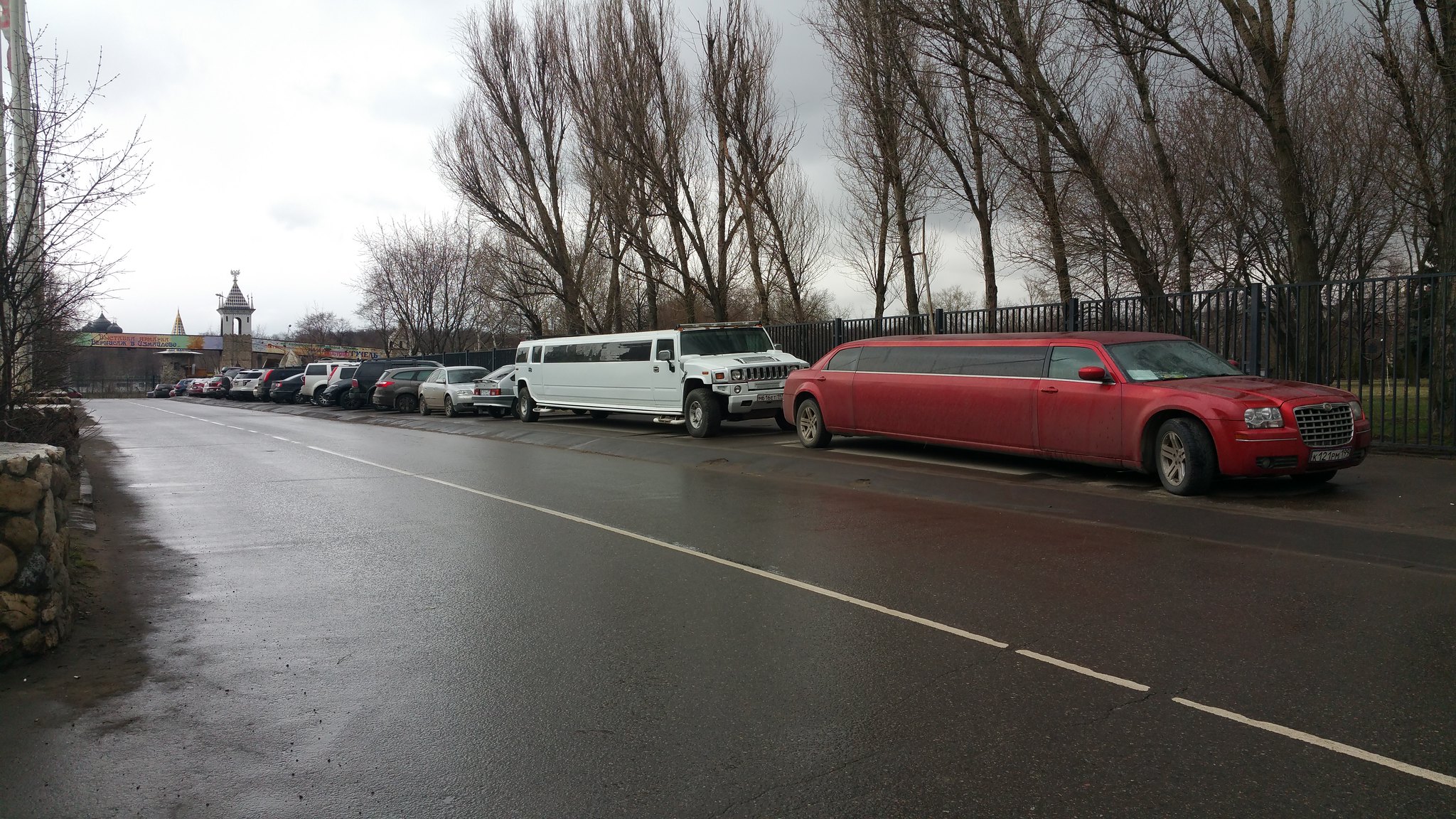The image depicts a wet, dark-paved street bordered by parked vehicles, dominated by two prominent limousines. The first, a striking red stretch limousine, is followed by a larger white Hummer limousine. The background reveals a group of slender, leafless trees, typical of winter, standing tall against a cloudy sky with patches of light and darker clouds. The street, marked by white lines, features a row of parked cars stretching into the horizon. On one side, a metal black fence runs alongside a grassy area. In the far distance, a quaint building with a triangular roof and cup-like columns, reminiscent of a church tower, adds a unique architectural element to the scene.